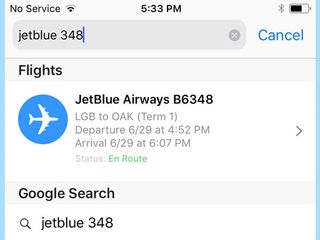**Detailed Caption:**
The image captures a screenshot from a cell phone displaying the top portion of a page with the device's toolbar. The status bar at the top indicates "No Service," the time is shown as 5:33 p.m., and the battery level is approximately 70%. The screenshot focuses on a Google search, where "JetBlue348" has been entered into the search box. The search results feature prominently, showcasing the details for flight "JetBlue Airways B6348." On the left side of the result, there is a blue circle containing a graphic representation of an airliner. To the right, the flight information is provided: the flight departs from Long Beach Airport (LGB) to Oakland International Airport (OAK), with a departure from Terminal 1 scheduled for June 29th at 4:52 p.m. and arrival on the same day at 6:07 p.m. The status of the flight is listed as "en route." Below this, there is a prompt to perform a new search, indicated by another search box with "Google search JetBlue348," reiterating the specific search terms used.